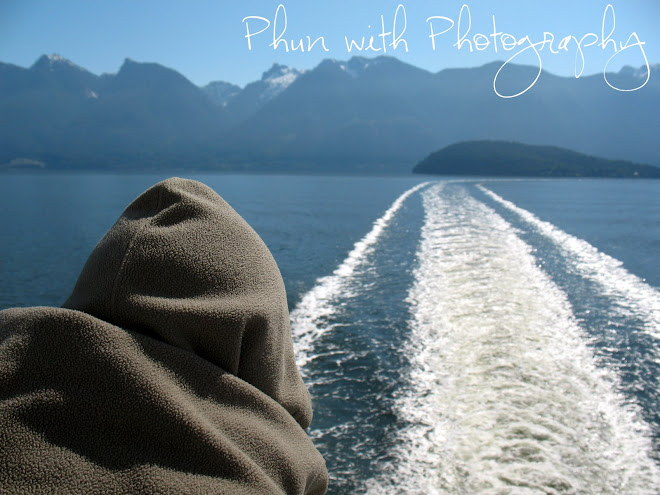The photograph captures a serene, blue, sunny day on a lake or ocean, framed by an expansive mountain range with a blue hue and snow-capped peaks. In the lower left corner, a person wearing a gray fleece hoodie with the hood up looks out from the back of a boat, steering or watching the trail of bubbles and waves created by the boat's motor. The boat leaves a long, winding wake stretching back toward a dark, elevated island visible on the right, suggesting the cold given the person's attire. At the top right of the image, in elegant cursive script, is the text "PHUN WITH PHOTOGRAPHY," indicating the photographer's playful style.